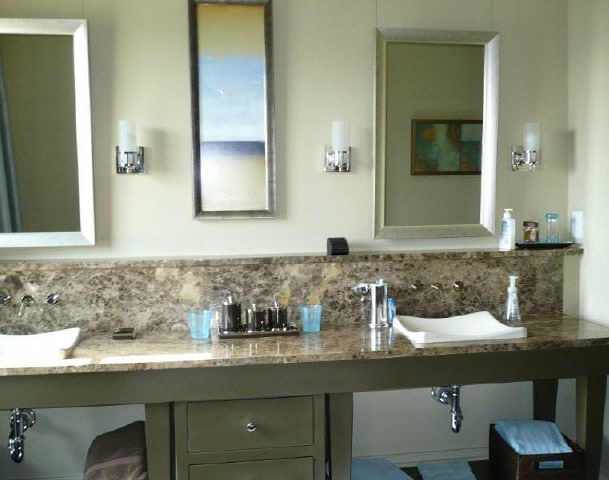The image captures a meticulously designed home bathroom featuring a his-and-hers layout with two separate white sinks positioned on the left and right sides of a long granite countertop. The countertop exhibits a polished surface of varied brown shades, providing a luxurious touch. Between the two sinks, ample counter space allows for shared use comfortably. Centrally placed on this counter is a small tray holding three dark-colored containers—possibly canisters or flask-shaped vessels—adorned with silver detailing. Flanking the tray are two light blue cups, adding a subtle contrast against the darker tones.

Underneath the countertop, the cabinetry is painted in a rich olive green, housing two visible drawers: a full one at the top and a partial one below. The cabinetry may conceal additional storage. Neatly folded towels are also placed below this counter, adding a practical element to the design.

Each sink is accompanied by its own sizeable mirror, with an additional rectangular mirror positioned centrally between them. Above these mirrors, three elegant sconce lights are mounted on the wall, providing harmonious and sufficient illumination. The overall design exudes both functionality and aesthetic appeal, ensuring a serene and efficient environment for morning and evening routines.